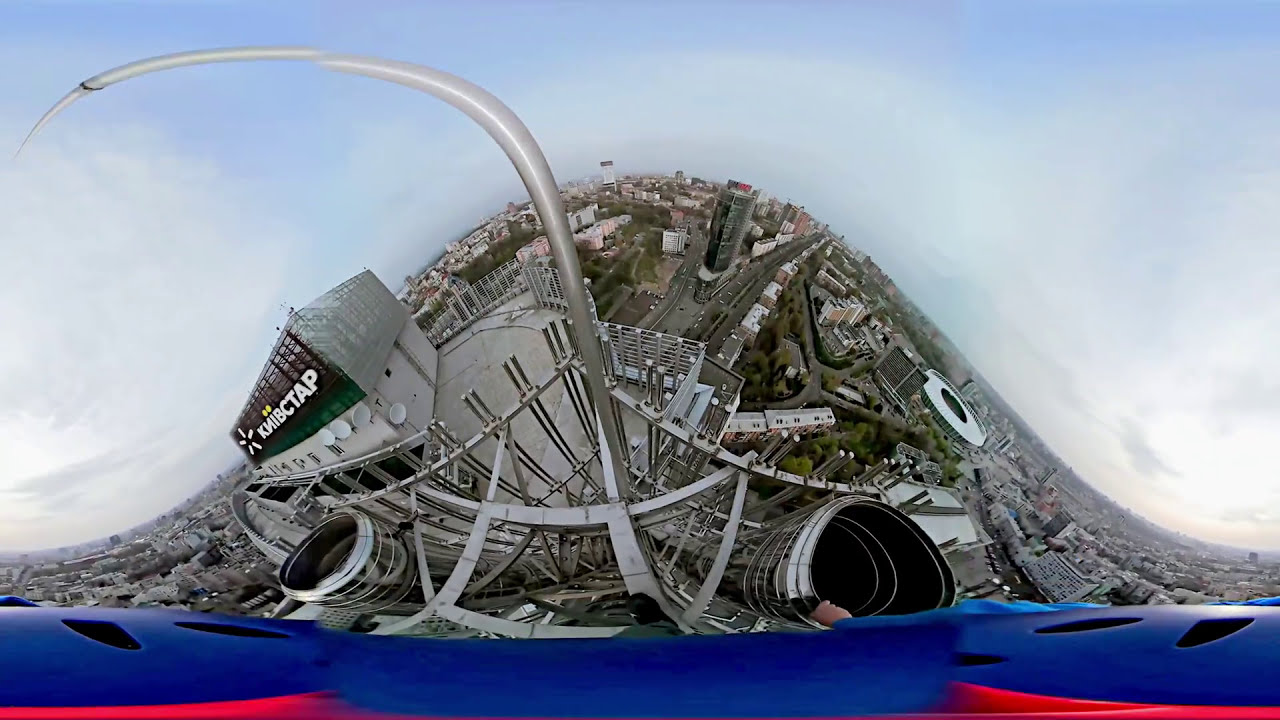This panorama, captured using a fisheye lens, presents a heavily distorted aerial view of a cityscape, likely taken from a daredevil's helmet cam perched atop a high construction rigging on a skyscraper. The view, from an extreme vantage point, transforms the city below into a bell curve illusion, tilting buildings and roads in a disorienting manner. The horizon, adorned with a light blue sky and feathery clouds, stretches out to the top and sides of the rectangular frame. Amidst the rigging and metal exhaust cylinders on the rooftop, a prominent white building structure stands out, featuring a green glass facade and a sign in Cyrillic, reading "КНИБСТАП" (KNIBCTAP), accompanied by a flower-like logo. This surreal perspective, juxtaposed with the intricate details of the rigging and the overarching sky, immerses viewers in a vertigo-inducing scene high above the city’s concrete jungle.